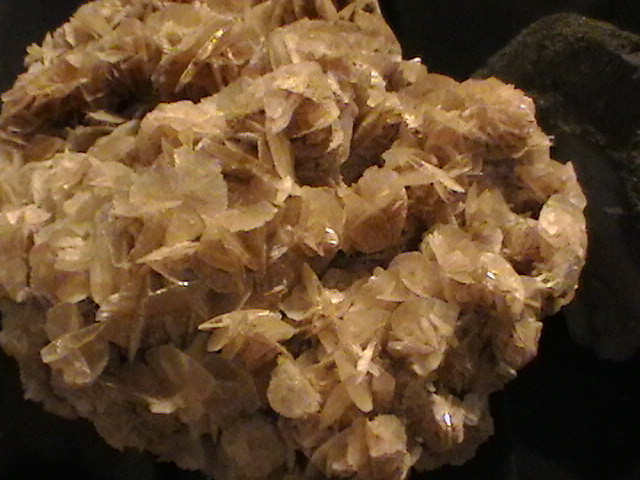The photograph depicts a centered, roughly four-by-four-inch image of an indistinct object, possibly a plant, bouquet, or a cluster of resin-like material. The main subject appears in a faded gold, light yellow, or brownish color, evoking the look of a withered bouquet or a textured, rock-like form. The object has a complex surface with several small, shiny elements reflecting light, resembling little wings or tightly packed structures. The background is predominantly black, adding to the unclear, grainy quality of the image, and a dark green shape is faintly visible on the right side. The overall image is vague and dark, leaving the object's exact nature uncertain.